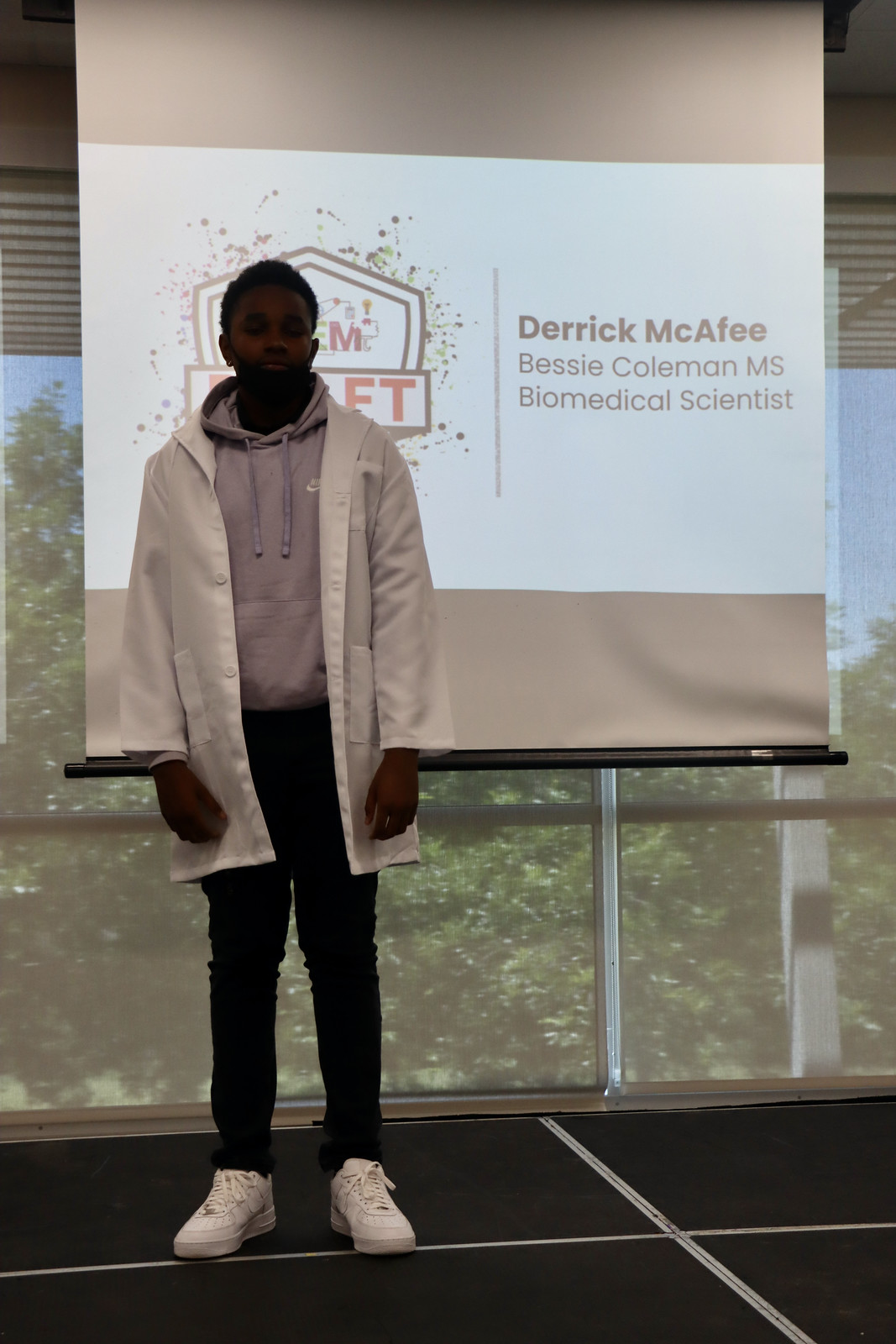The vertically aligned rectangular image features a young man standing confidently. He is dressed in a white lab coat over a gray hoodie, paired with black pants and white tennis shoes. He has very short black hair and dark skin. Behind him, a screen displays the name "Derek McAfee," followed by "Bessie Coleman, M.S." and "Biomedical Scientist." Partially obscured by his body, there's a logo to the left. The backdrop includes a large wall depicting an outdoor scene with a blue sky and lush green trees. The black floor he stands on is adorned with intersecting white vertical and horizontal lines.